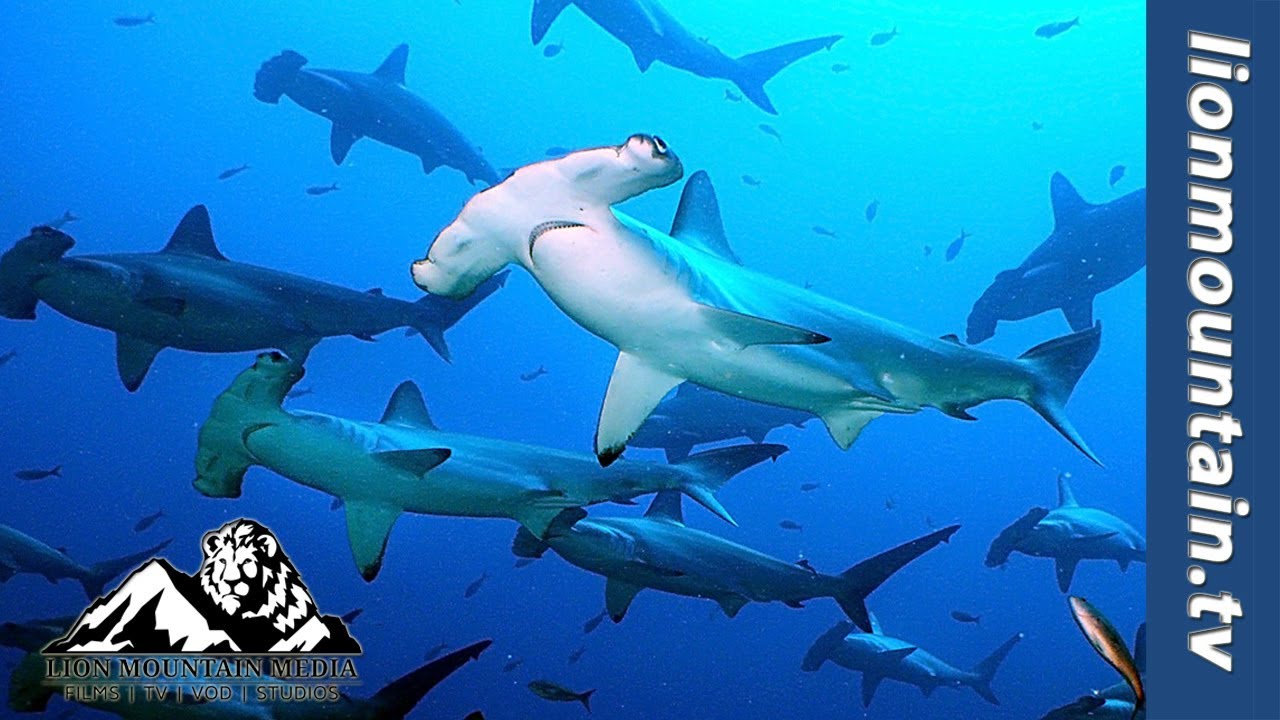The image displays an underwater scene dominated by a school of hammerhead sharks swimming in blue waters. Most of the sharks are cast in shadow, except for one prominent shark that stands out with its cartoon-like, expressive eyes and a semi-circular smile. This shark features a white underside fading into gray-green hues. Surrounding the sharks are numerous small fish, with their count appearing to be around a dozen. 

In the background, towards the bottom left corner, there's a black and white logo depicting a lion on a mountain, and beneath it is the text "Lion Mountain Media Films TV VOD Studios." On the right side of the image, a vertical blue stripe contains white text that reads "lionmountain.tv." This cohesive blend of marine life and commercial branding creates a captivating and detailed visual narrative.